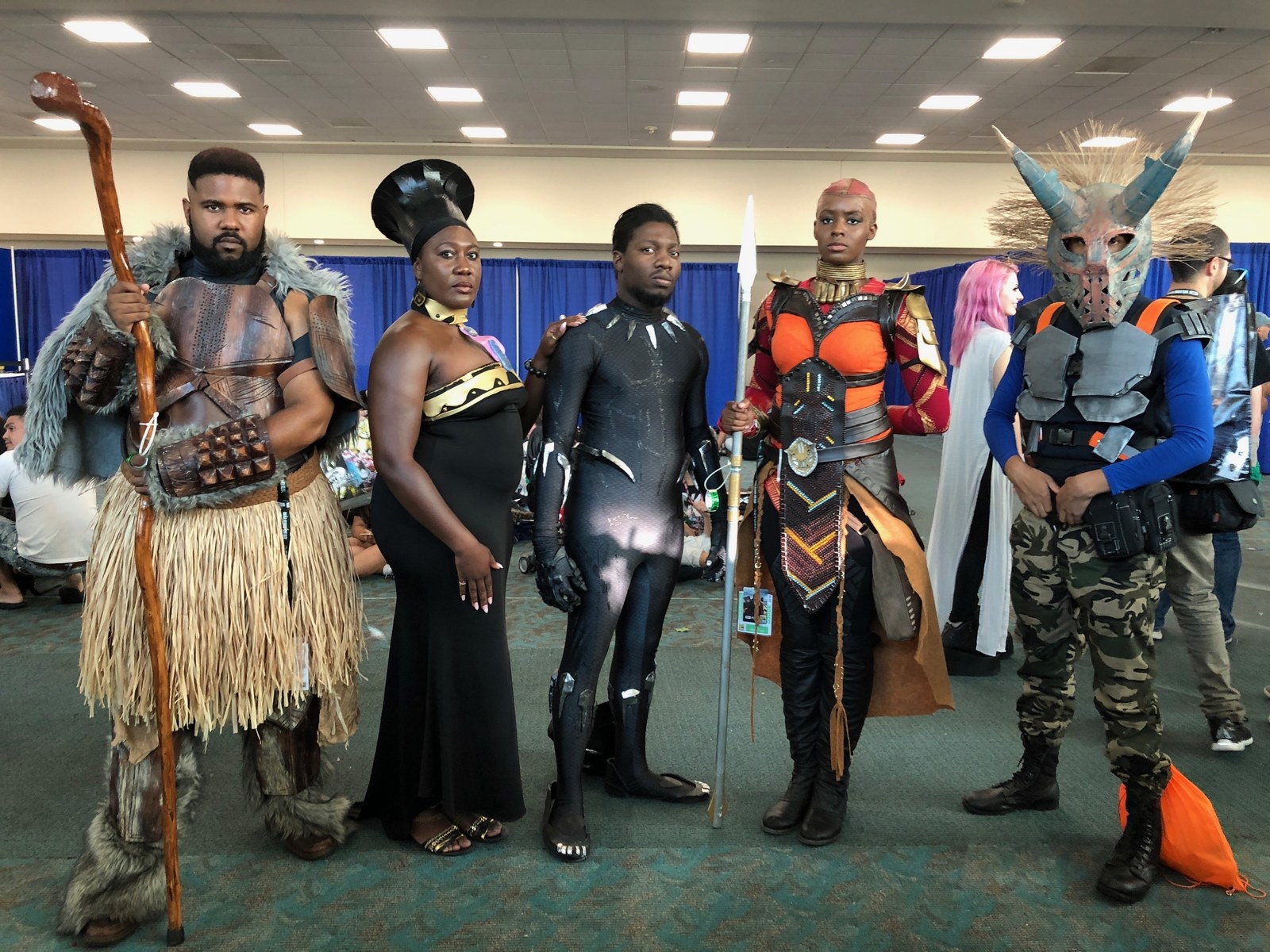The image is a detailed photograph of a diverse group of cosplayers, most likely attending a convention such as Comic-Con, dressed as characters from the "Black Panther" movie. The group consists of two women and two men, all of whom appear to be African-American. In the foreground, the man on the left is donning a beige hay skirt, a gray fur cape, and matching fur boots, reminiscent of an attire from the Golden Tribe. Next to him stands a woman in a striking black dress with gold accents across the chest and a tall, elegant black hat. The second man is clad in a black suit that resembles the tight-fitting costume of the titular character, albeit somewhat awkwardly fitted to his body. The second woman is dressed in an orange outfit paired with black pants, suggesting a character of significant importance, potentially Queen Ramonda. Standing out among them is a white man in the far right wearing a costume adorned with large horns, adding a layer of fantasy to the scene. 

In the background of the convention-like setting, a woman with vibrant purple hair and a white tunic can be seen, along with other indistinct objects on the blue-draped floor. This detailed setting and the distinctive costumes vividly capture the essence of a lively cosplay event dedicated to the cultural phenomenon of "Black Panther."